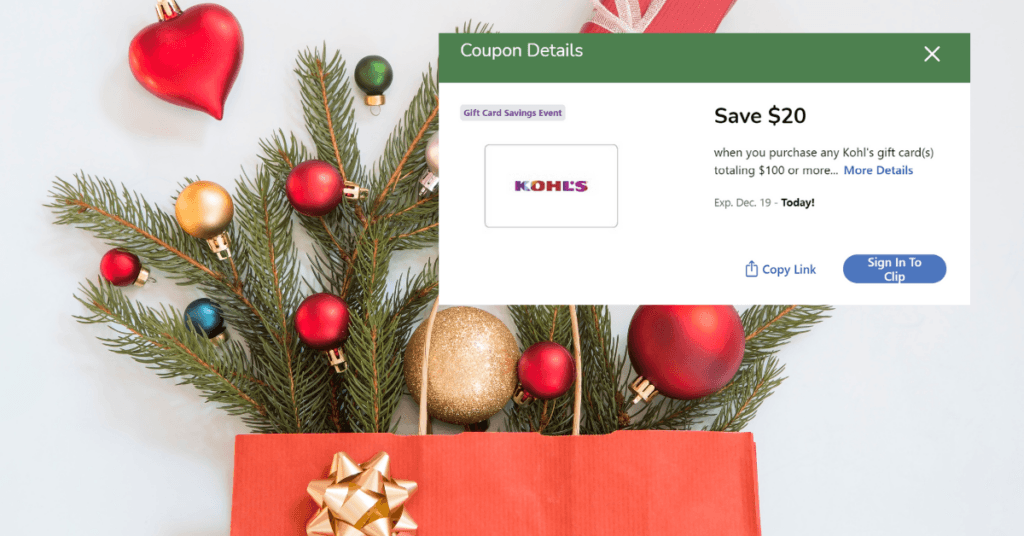Holiday Advertisement for Kohl's: 

Set against a sophisticated gray background, this festive advertisement showcases a red gift bag adorned with a luxurious gold bow, artistically laid flat on a table. Emerging from the gift bag are elements reminiscent of a beautifully decorated Christmas tree: five to six lush fir tree branches, and a variety of vibrant Christmas ornaments. Among the ornaments, you’ll find several classic red balls, a charming red heart-shaped ornament, a dazzling gold ball, a tranquil blue ball, a lush green ball, a sleek silver ball, and one glitter-encrusted ball, adding extra sparkle to the scene.

In the foreground, a prominent green pop-up box with a white font and a green band across the top draws your attention. It reads "Coupon Details." Below this heading, within a stretching white rectangle, the Kohl’s logo is prominently displayed. The offer reads: “Save $20 when you purchase any Kohl’s gift cards totaling $100 or more." This enticing deal, urging customers to buy $100 worth of Kohl’s gift cards to receive an additional $20 gift card, is accentuated by a time-sensitive note indicating the offer expires on December 19. This ad perfectly captures the holiday spirit while presenting a compelling limited-time offer.